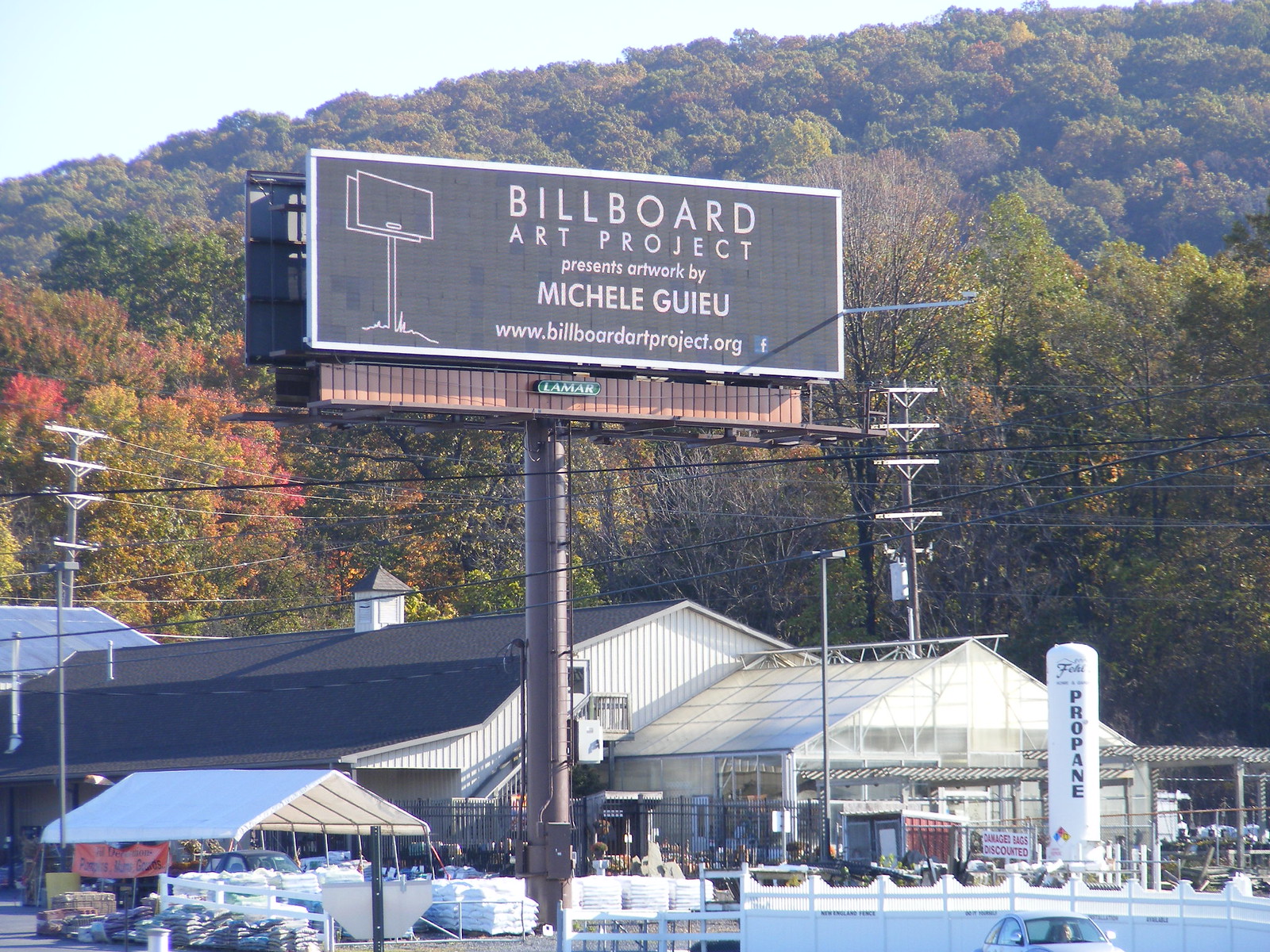The daytime color photograph captures a billboard prominently displaying white text on a black background, framed in white. The text reads "Billboard Art Project presents artwork by Michelle Guieu" (spelled G-U-I-E-U), alongside the website "www.billboardartproject.org" and a Facebook icon. The billboard is positioned above a series of power lines and overlooks a building with a sloped, dark-colored roof, which appears to be a home and garden store. This store features a greenhouse, a large propane tank, and stacks of materials such as mulch in the parking area. The surrounding landscape includes a wooded hill partially covered in colorful autumn foliage, featuring hues of yellow, red, and green. Additional structures below the billboard include brown shed-roof buildings, a barn, a silo, and outdoor tent structures.